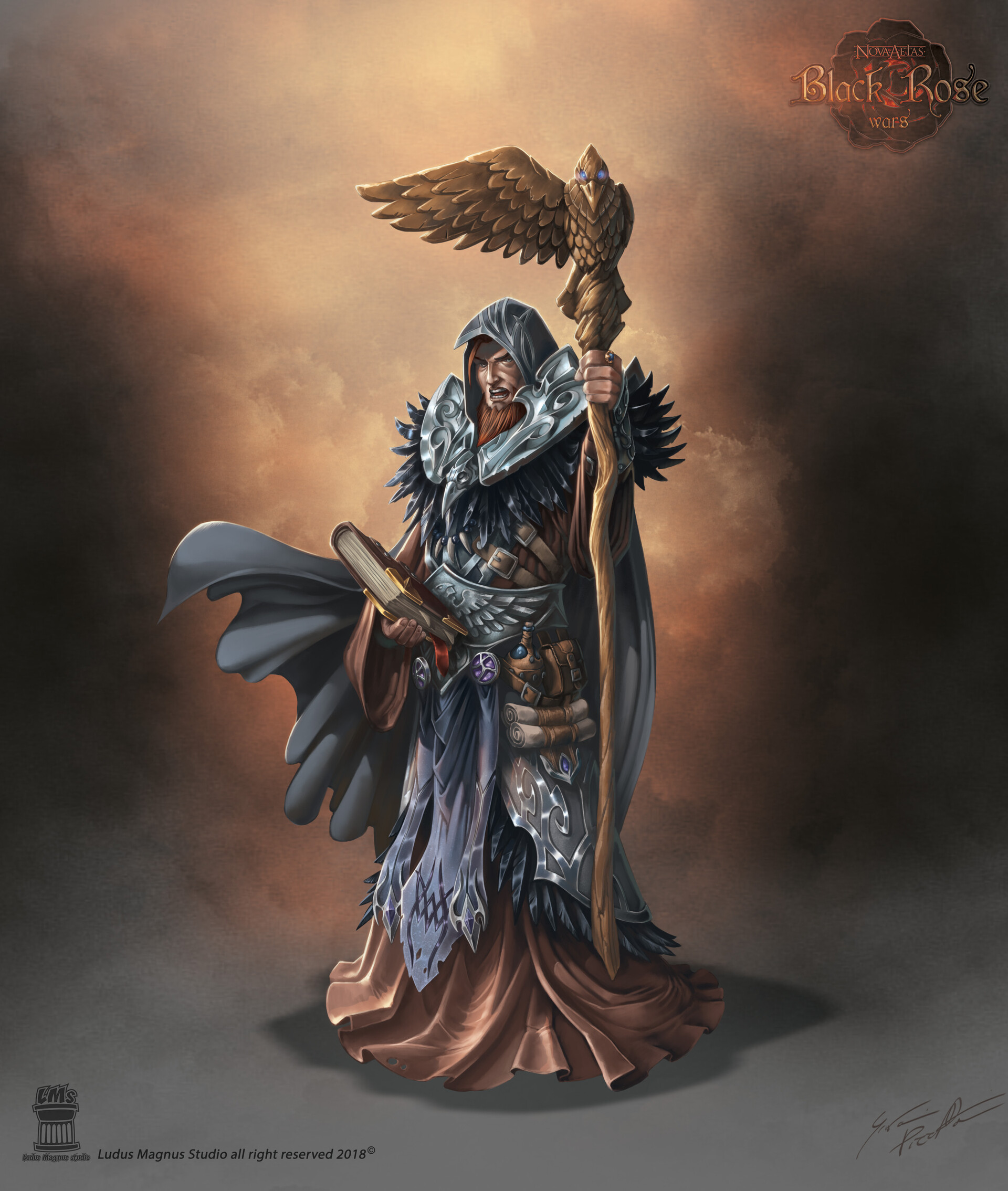The image is a detailed color illustration in a fantasy style, featuring a character that resembles a warlock or mage from a video game. The character stands against a smoky, orangish-gray background with a lighter tan hue emanating from behind, creating an illusion of backlighting. In the upper right corner, the words "Nova Atlas Black Rose Wars" are visible as a watermark.

The figure is adorned in armor with large metal shoulder elements, accentuated by black feathers underneath. He wears a helmet, a gray cape flaring out to his left, and numerous straps across his chest. His brown robe extends downward, blending with the metal elements. A significant metal belt, shaped somewhat like a wing, cinches his waist.

In his right hand, he holds an intricately detailed book, and in his left hand, he grips a tall staff topped with a sculptural bird that has gem-like blue glowing eyes and one outstretched wing. The character's expression is stern, with a brown beard enhancing his grim demeanor.

At the bottom right corner of the image is an artist's signature, though it is not legible, and the bottom left corner contains the text "Ludus Magnus Studio, all rights reserved, 2018," accompanied by a copyright symbol.